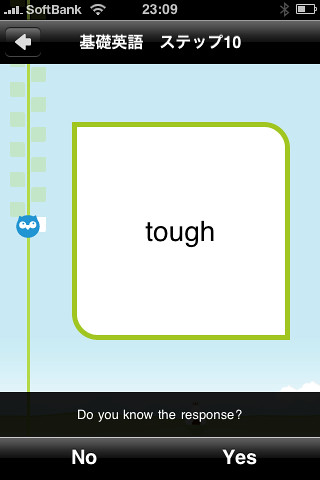This image is a screenshot of a phone app, displayed in an interface primarily in Japanese or another Asian language. At the top left of the screen, the status bar shows "SoftBank" as the carrier with 4 out of 5 bars for signal strength, a WiFi icon centered at the top, and the time "23:09," indicating it's almost midnight. On the top right, there's a greyed-out Bluetooth icon and a battery icon showing about 45% power, albeit without a numeric percentage. The app screen itself features a back arrow button on the top left, some Asian text in the middle, and the number "10" on the right. The main section of the app has a white tile card with black text displaying the word "tough." To the left of this card is a blue owl icon. The background of the screen is light blue. At the bottom of the card, a prompt reads, "Do you know the response?" followed by "no" and "yes" options. This appears to be part of an English learning app.